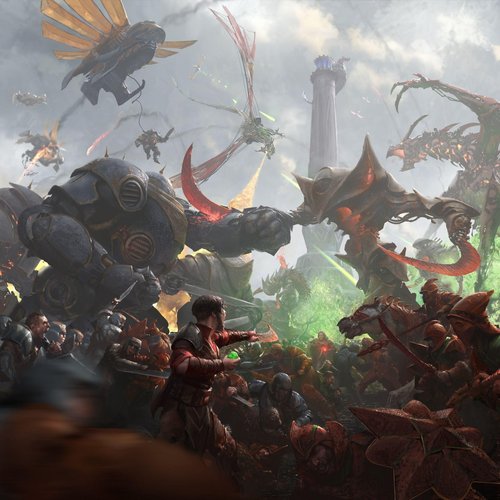This detailed and vibrant scene is set in a large-scale fantasy and sci-fi battle, reminiscent of climactic video game concept art or anime action sequences. At the heart of the image is a central figure—a human, clad in a red combat outfit with short brunette hair, crouching and pointing upwards with arms stretched out aggressively, ready to engage in the fierce conflict. The backdrop features a stormy gray sky, with a foreboding dark gray tower rising in the mid-right, adding to the dramatic tension of the scene.

Surrounding the central character is a chaotic melee of combatants, all similarly dressed in dark reddish and gray tones, seemingly converging on the focal figure. Adding to the mayhem, several monstrous and mechanical entities dominate the battlefield. On the mid-left side of the screen, a colossal dark gray robot with imposing arms looms menacingly, while on the mid-right, a fierce dragon with gray scales and red accents interweaves through the battle, some of its draconic peers spewing flames from their mouths.

The sky teems with additional mythical creatures, including dragons and other flying beasts, enhancing the epic scope of the confrontation. The overall scene is a thrilling, high-stakes clash, evocative of legendary cinematic battles, with a mix of humans and fantastical beings, poised in a dramatic standoff amid a chaotic and visually striking environment.